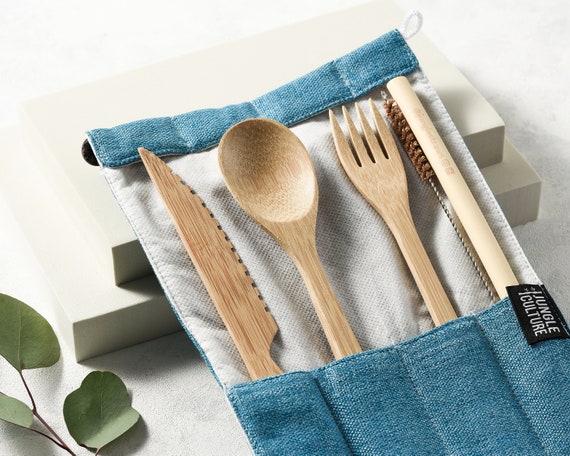This is a color photograph featuring a set of wooden utensils neatly arranged in a light blue, cloth-like fabric holder with individual sleeves for each item. The holder displays a black tag with white writing that reads "Jungle Culture." From left to right, the holder contains a wooden knife with its blade pointing to the right, a wooden spoon, a wooden fork, a reusable drinking straw, and a bottle brush with brown bristles. This holder is placed on a small pedestal made up of two white rectangular blocks, giving it an elevated display against a mostly light gray background. To the bottom left of the image, a sprig with three round green leaves adds a natural decorative touch. The setup appears to be designed for a catalog or advertisement photo, emphasizing the eco-friendly and stylish presentation of the utensils.